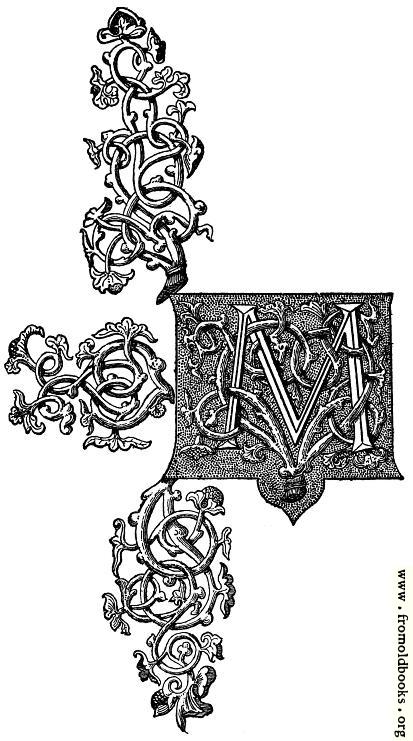The image is a meticulously detailed, black and white collage featuring intricate filigree illustrations that resemble tangled vines sprouting various leaves and flowers. At the center of the collage, a prominent letter "M" entwined in the filigree appears to be emerging from a shield-like structure. The entire composition, possibly hand-drawn or digitally produced, conveys an elaborate, tattoo-art aesthetic. The artistic quality suggests it could be akin to chapter markers or ornate decorations in old manuscripts. Additionally, along the right-hand side of the image, the URL "www.fromoldbooks.org" is displayed vertically, reinforcing the impression that this artwork originates from or is inspired by historical book illustrations.